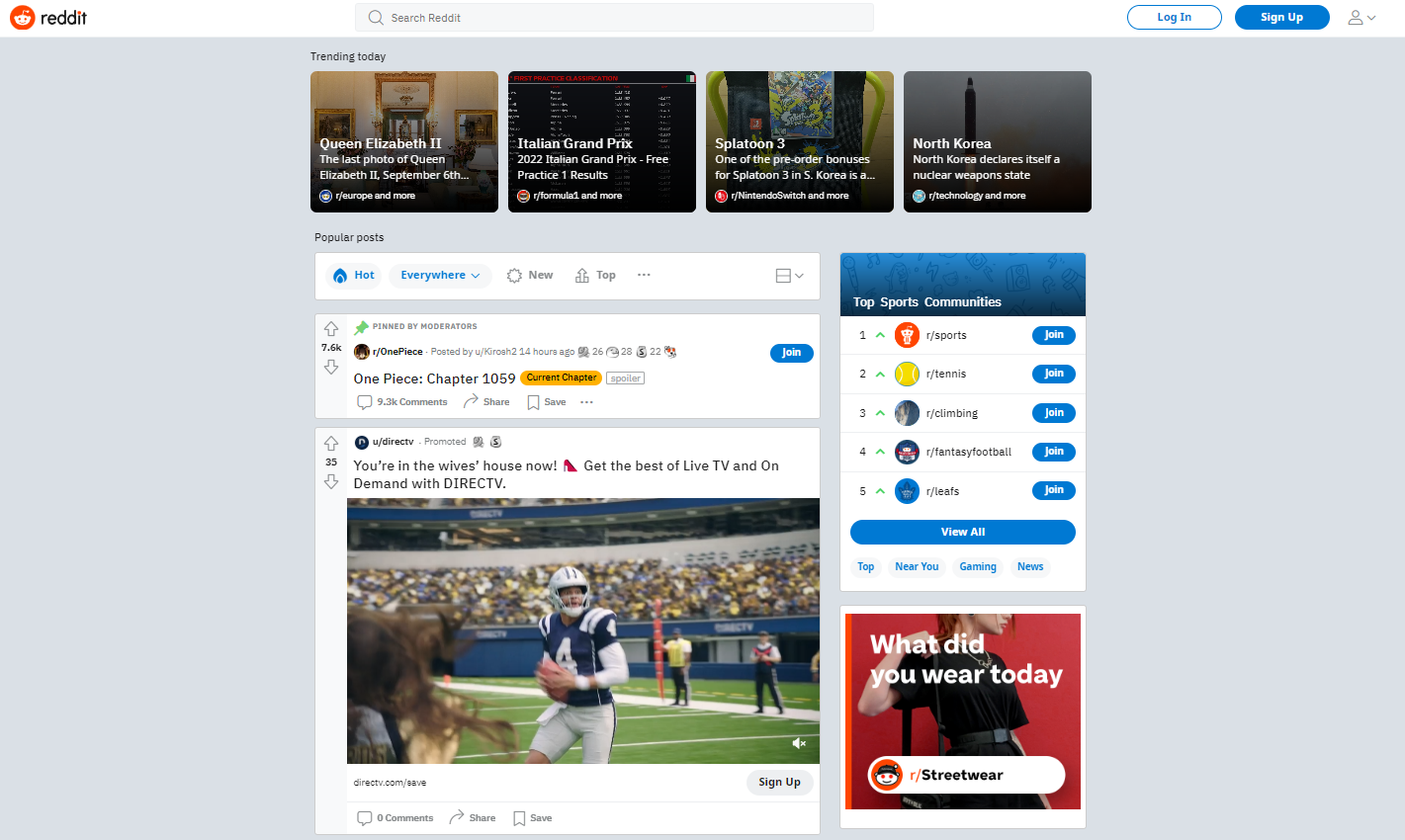A detailed screenshot of the Reddit homepage is presented. In the top left corner, the Reddit logo is visible. Centrally positioned is a search box with the placeholder text "Search Reddit" in light grey letters. On the far right, there is a button outlined in light blue that says "Log In" in the middle, also in light blue. Adjacent to it is a light blue button with white text saying "Sign Up". In the far right corner, there is a user icon with an accompanying drop-down menu.

The page’s background is grey. Horizontally arranged at the top are four thumbnails, with the leftmost one displaying the text "Trending Today" in the top left corner. Each thumbnail showcases a different story headline. Below the thumbnails, in light grey text, it says "Popular posts".

Beneath this, there is a white rectangular bar with several options: "Hot", a drop-down box titled "Everywhere" (currently selected), "New", and "Top". To the right of "Top" are three dots indicating additional options, and further to the right is another drop-down box allowing selection between list view or page format.

Lower on the page is a white post box marked "Pinned to the top". An option to "Join" is on the right side. Below this, there is a "Promoted Post".

On the right side of the page is a tall rectangular column titled "Top Sports Communities", listing the top five sports-related groups. Each group has a "Join" button on the right and is numbered on the left, starting with #1 as "sports", #2 as "tennis", and so on.

At the bottom right is a small box with the text "What did you wear today?" and features a photo thumbnail beneath the text. There is also a banner that reads "Our Streetwear".